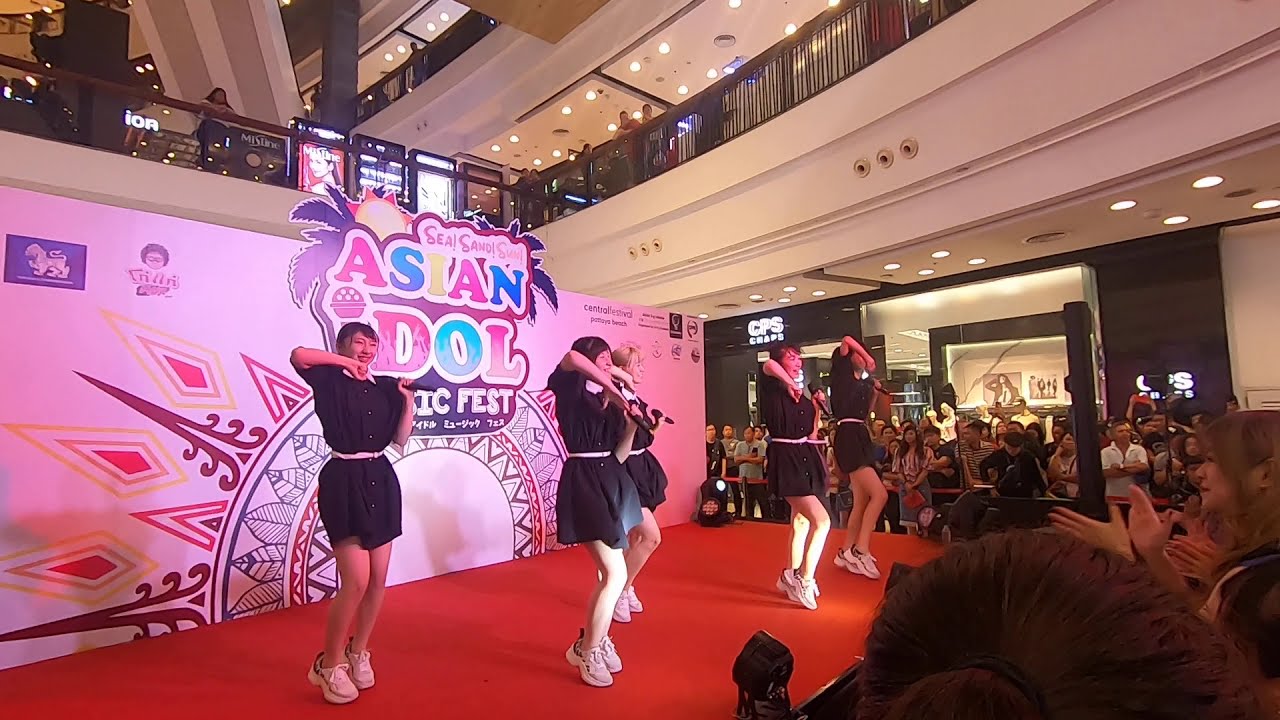The image depicts an energetic scene inside a bustling shopping mall, showcasing a vibrant dance performance. Center stage, which is adorned in red, features five Asian women dressed uniformly in black dresses with white belts and white sneakers. Each performer holds a microphone and they are captured in a synchronized dance pose. A large pink backdrop behind them prominently displays the text "Asian D-O-L Music Fest." The audience, a diverse group not primarily composed of Asian onlookers, is intently watching the performance. Spectators are seen applauding and enjoying the show from multiple vantage points, with crowds gathered on both the ground level and the mall's two upper floors, peering over railings. The mall's second floor, right above the performance area, is especially crowded with viewers, and even higher up, a few people are visible on the third floor, also engrossed in the performance. Toward the right side of the image, there's a storefront labeled CPS, adding to the detailed indoor mall setting.